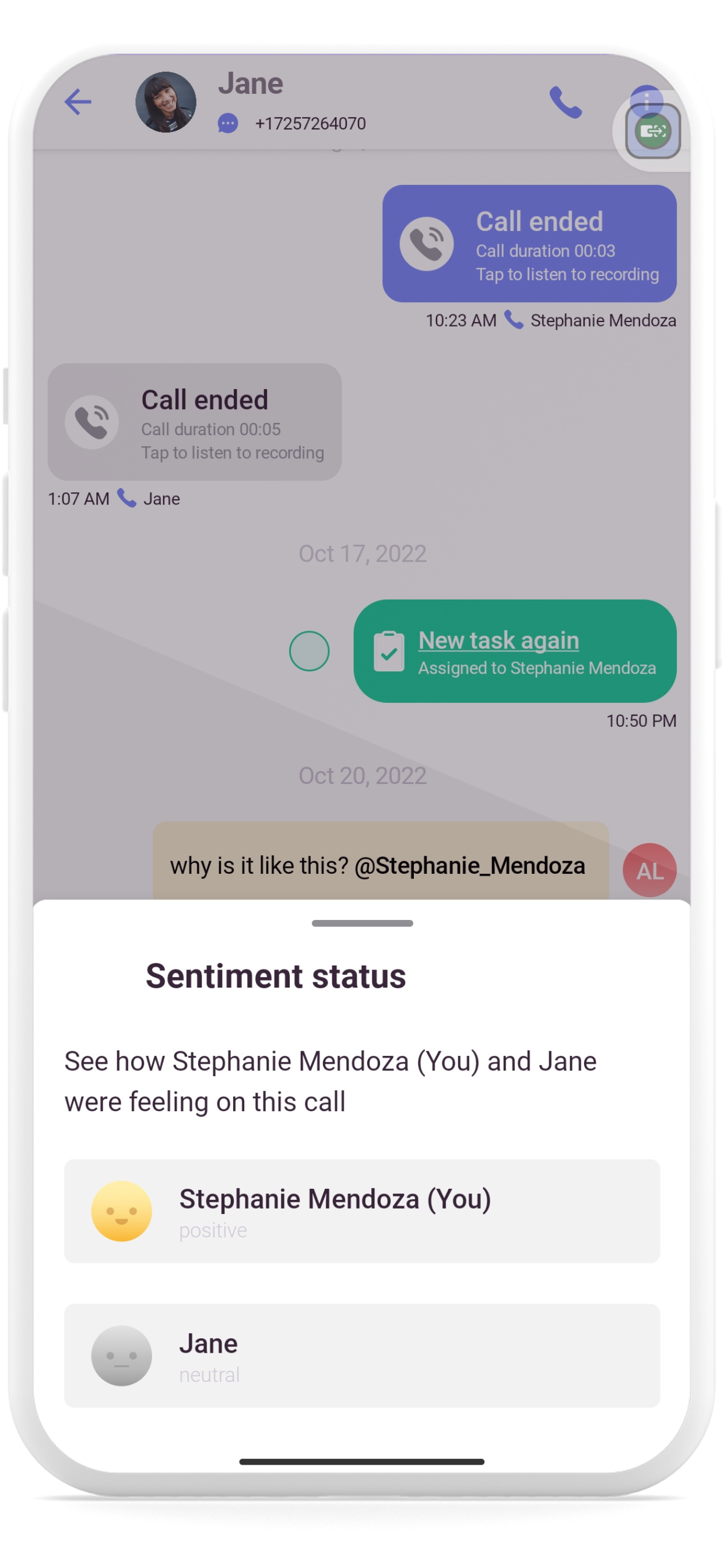The image displays a cell phone screen, with the top portion appearing grayed out due to a pop-up box at the bottom. The phone's physical features, including three buttons on the left side and one button on the right side, are visible. At the bottom of the screen, a gray line sits centrally above a text box that reads, "Sentiment Status." The text continues with, "See how Stephanie Mendoza (you) and Jane were feeling on this call."

Below the text for each person’s sentiment, Stephanie Mendoza’s status shows a yellow smiling face icon labeled "positive." In contrast, Jane has a gray face icon with a straight-line mouth, labeled "neutral." The background of the image includes additional information such as "call ended," the duration of the call, and specific details regarding Stephanie Mendoza and Jane. It also mentions a new task assigned to Stephanie Mendoza, which says, "Why is it like this?" along with her name beside the task.